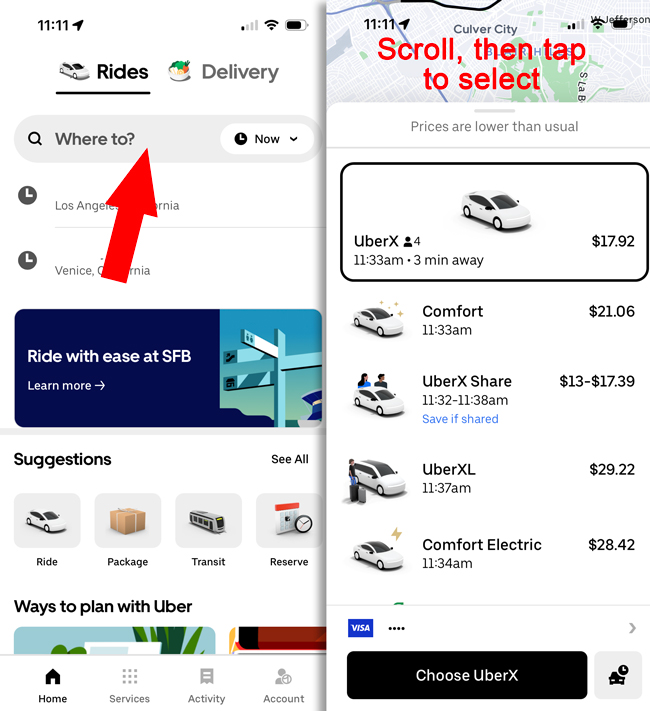The image consists of two overlapping screenshots displayed on a white background. The first screenshot prominently features the text "RODS delivery," with the word "RODS" underlined in black. There is a question mark following the phrase "where to," positioned next to a magnifying glass icon. Below that, there is the word "Now" enclosed within a white oval, next to a clock icon. The text "Loss in" appears cut off, followed by fragmented words "events V" and “I Venice.” Additionally, there is a red upward-pointing arrow directed towards the "where to" oval and the phrase "rod with ease at SFB." The bottom of the screenshot includes informative prompts such as "learn more," "suggestions," "see all," and options related to "rod package transit" and "reserve ways to plan with Uber." At the lower edge, there is a navigation bar with "Home" highlighted in black, while other options like "services," "activity," and "account" appear in gray.

The second screenshot shows a map centered on Culver City, highlighted in red. A prompt instructs users to "scroll, then tap to select" while noting that "prices are lower than usual."